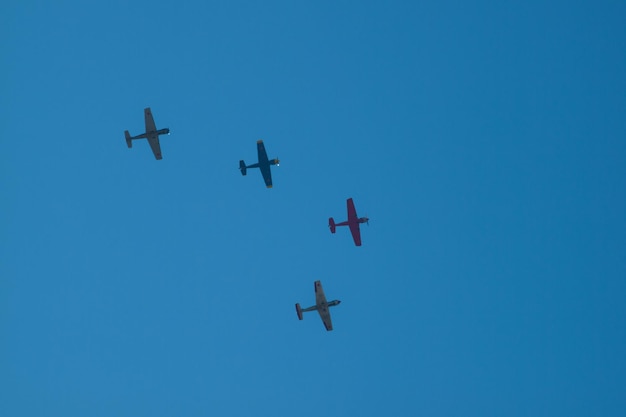This color photograph captures four World War II-era propeller planes flying in a V formation against a clear, cloudless blue sky. The planes, blurred and silhouetted in the distance, appear as black shapes with discernible propellers and tails. Flying from left to right and slightly off-center toward the bottom of the image, the formation features one lead plane with three others following: two on the top part of the V and one below, slightly trailing. The lead plane is said to be red, while those trailing include a blue, a yellow, and another yellow aircraft, though such colors are not distinct in the silhouetted presentation. The minimalist backdrop emphasizes the historic planes’ form and positioning within the expansive, evenly shaded blue sky.